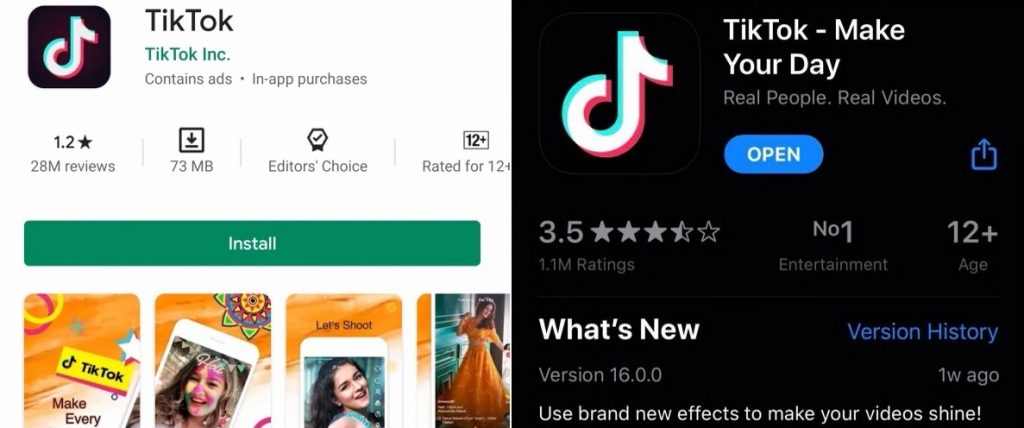This image showcases the TikTok app's download page. On the left, there's a white square featuring the TikTok icon with text that reads, "TikTok, TikTok Inc. Contains ads and in-app purchases." Below that, it shows a rating of 1.2 stars from 28 million reviews. A download symbol next to the size "73MB" is displayed, followed by an icon indicating "Editor's Choice." To the far right is a square indicating the app is rated for ages 12 and up.

Below this primary section is a prominent green "Install" button, and beneath it are four separate promotional images. The first image reads "TikTok Make Every," while the next features a female with her face tinted pink. The third image includes the text "Let's Shoot" along with a picture of a different female, and the final image shows a female in a long orange dress dancing.

To the right, another section showcases a black background with "TikTok Make Your Day, Real People, Real Videos" and the TikTok icon. A blue button labeled "Open" is also present, accompanied by an upload arrow symbol. This part of the page displays a 3.5-star rating from 1.1 million ratings, the label "No. 1 Entertainment," and an age rating of 12+. The "What's New" section includes a clickable "version history" in blue, indicating version 16.00 was updated one week ago.

At the very bottom, a statement encourages users to "Use Brand New Effects to Make Your Videos Shine."